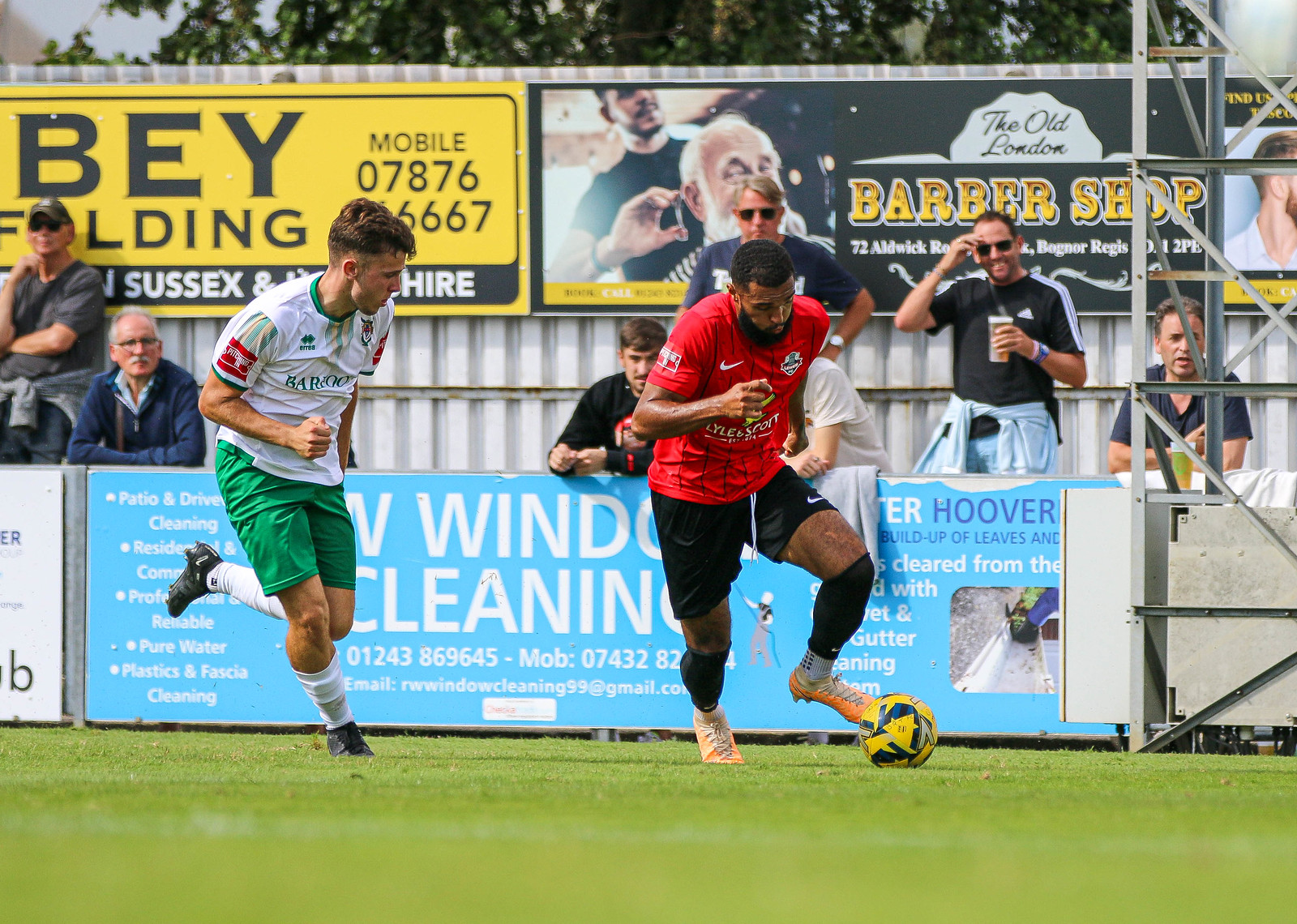The photograph captures an intense moment during a live soccer match on a green field. Centered in the frame, two players compete for a yellow and blue soccer ball. The player on the right, who has a beard and looks like a black man, is dribbling the ball while wearing a red jersey, black shorts, black shin guards, and white and orange shoes. His opponent, on the left, is running after him, dressed in a white jersey, green shorts, white socks, and black shoes. Behind the players, the sideline is lined with advertisements. A prominent teal banner with white writing advertises a window cleaning service, showing partial contact details like a phone number and email. Additionally, bullet points on the banner mention services such as patio and driveway cleaning and professional reliability. Further behind, spectators, consisting of adult males of various ages, are visible watching the match from behind another barricade adorned with more advertisements. These include a yellow banner with partially visible text and a charming ad for "The Old London Barber Shop" at 72 Orwick Road, Bognor Regis, featuring an image of an old man getting his hair cut.